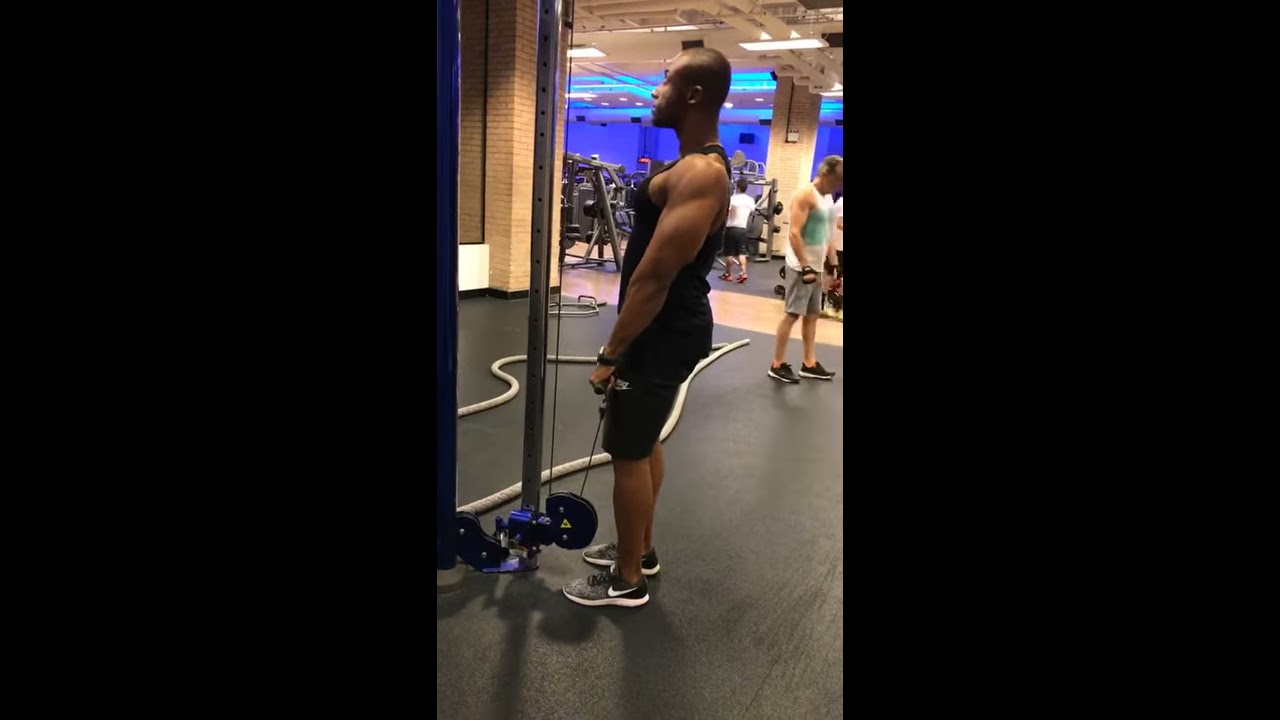In the gym, amidst various high-end workout equipment and several patrons engaged in different activities, stands a muscular man of African descent. The centrally positioned photograph shows this man, in sharp focus, facing his left profile. Clad in a black tank top, black shorts, and Nike sneakers, he appears deep in concentration, his eyes closed. His close-shaven black hair adds to his determined look. The man is grasping a bar attached to a pulley machine, seemingly preparing for a set of pull-downs or curls. The gym's sophisticated ambiance is accentuated by the gray padded flooring, brick walls, and blue lighting. Weighted gym ropes rest in the background, adding to the dynamic environment. Other individuals are seen utilizing various equipment, contributing to the vibrant atmosphere of this well-equipped fitness center.